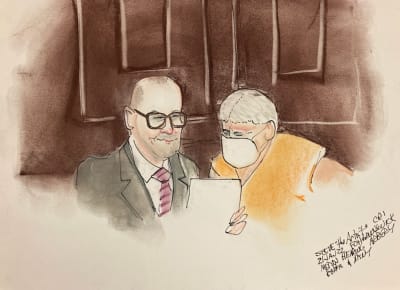The image depicts a detailed sketch of a courtroom scene featuring two main figures in the foreground, set against a background of browns, dark browns, and subtle whites. The background, likely depicting a formal wall finish, adds to the courtroom atmosphere. On the left side of the image is a balding man, likely the lawyer, characterized by his black-rimmed glasses and attire consisting of a gray suit jacket, white shirt, and a tie with pink and black stripes. He appears to be holding a piece of paper in his left hand, which he is showing to the other person. The person on the right, presumed to be the defendant, wears an orange, sleeveless shirt or possibly a prison jumpsuit and a white COVID-style face mask. He has short gray hair. Both individuals are focused on the document the lawyer is holding. Surrounding them, there is a cloudy imprint effect that adds to the sketch's illustrative nature. Additionally, some unreadable writing is present at the bottom right of the image.